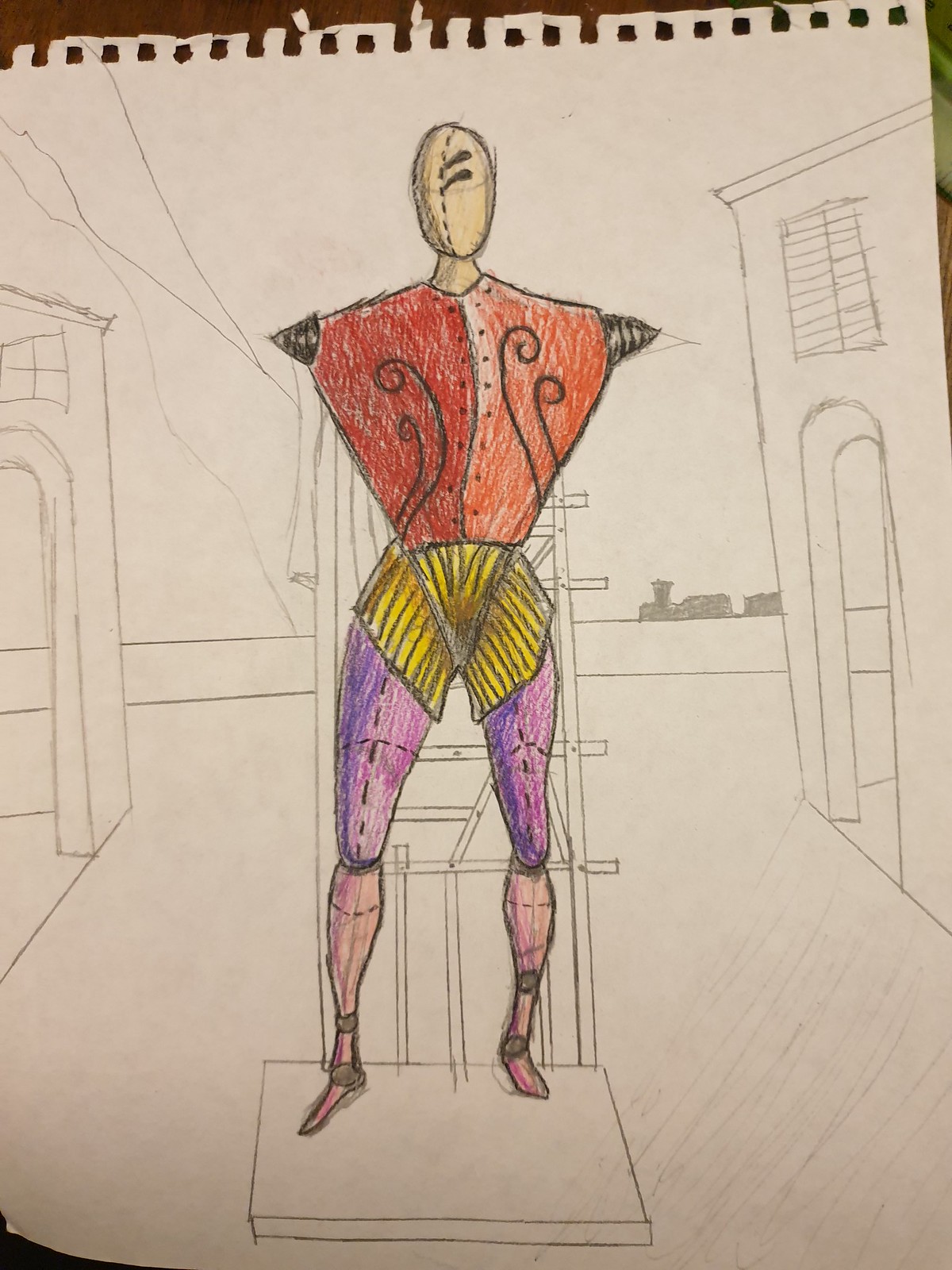A detailed sketch in a sketchbook captures an enigmatic scene in a town setting, flanked by faint outlines of buildings on both the left and right sides. The focal point of the drawing is a peculiar figure standing on a platform with visible supports behind it. This figure, devoid of eyes, nose, or mouth, suggests the appearance of a statue, mannequin, or maybe even a robot in the making. The figure's anatomy is unconventional, with spiraled shapes instead of arms, and a body segmented into distinct color zones— a red torso adorned with curved designs, a yellow hip area, purple thighs, and pinkish calves leading down to its feet. The detailed platform hints at the figure being displayed or constructed, adding a layer of mystery to the artistic depiction.